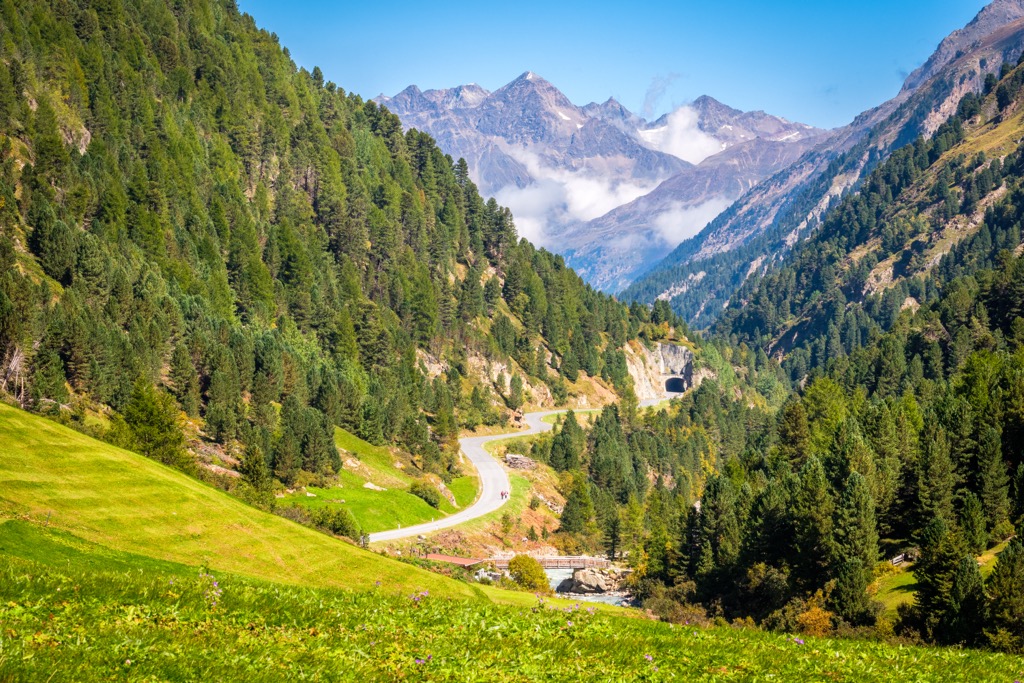The image captures a breathtaking mountain landscape, providing a blend of natural beauty and human exploration. In the distance, majestic blue-gray mountains dominate the horizon, some still dusted with remnants of snow and possibly shrouded in light fog or steam, evoking a sense of tranquility. These mountains transition to a slightly bluer hue as they meet the lush, green forested areas at lower elevations. The foreground is a vibrant tapestry of green grass, interspersed with patches of darker green and small streaks of orange, creating a rich palette of colors. A central pathway, potentially a road, weaves its way through the landscape, flanked by dense green trees. Along this road, two travelers can be seen making their way by foot. The pathway leads to a distant tunnel and crosses a bridge over a body of water, adding elements of adventure and human presence to the serene natural setting. The overall scene, likely captured in early spring, showcases a harmonious blend of untouched wilderness and subtle human activity.